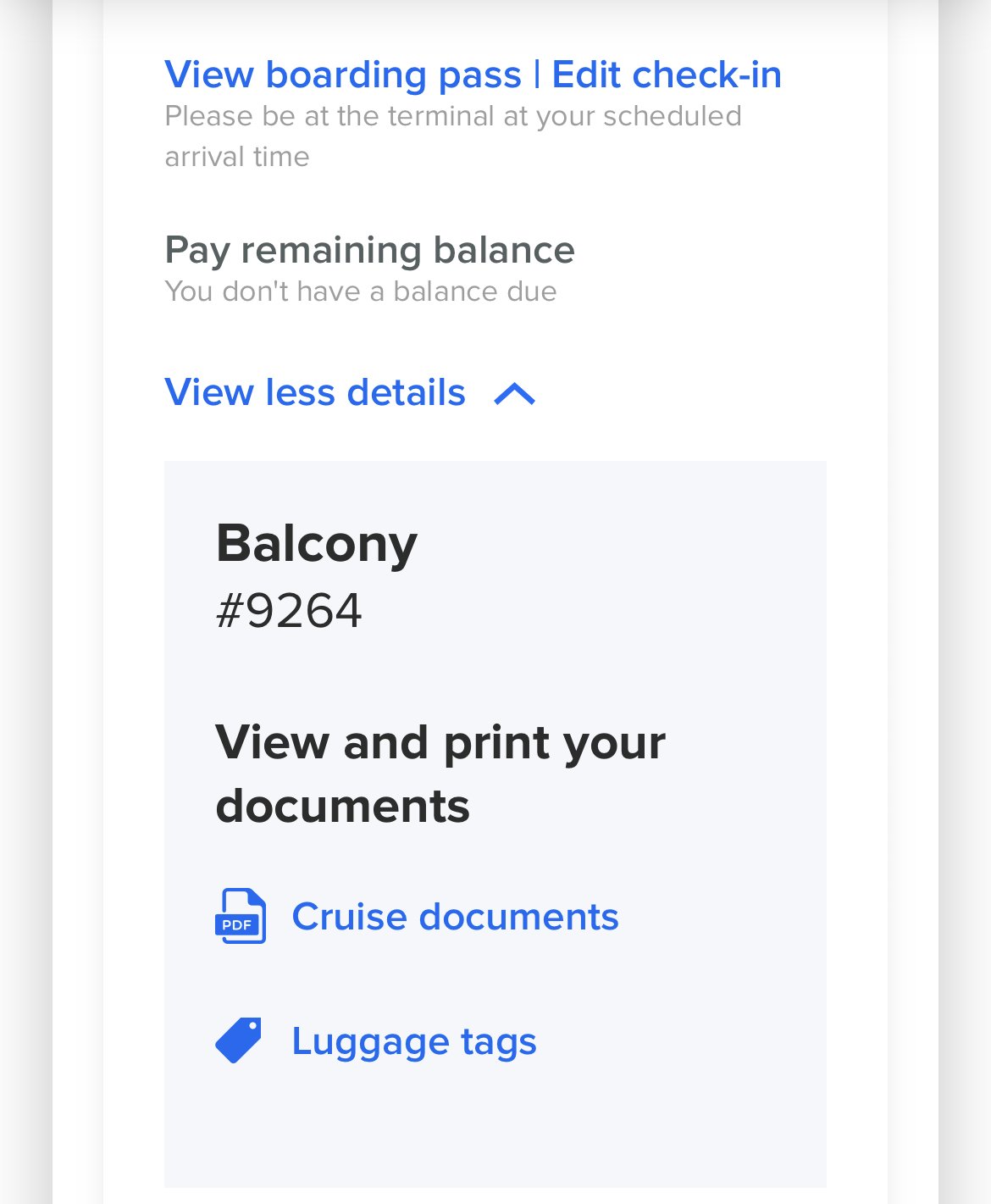The image displays a digital boarding pass for a cruise. The interface offers several options in clear black and gray text: "View Boarding Pass," "Edit Check-In," and "Pay Remaining Balance" (although it appears there is no outstanding balance). The specific seating assignment is indicated as Balcony, cabin number 9264. Initially, this setup might seem reminiscent of an airplane boarding pass, but it is, in fact, for a cruise. The interface also includes options to view and print crucial cruise-related documents, such as cruise documents and luggage tags, ensuring all necessary preparations are covered for the voyage.